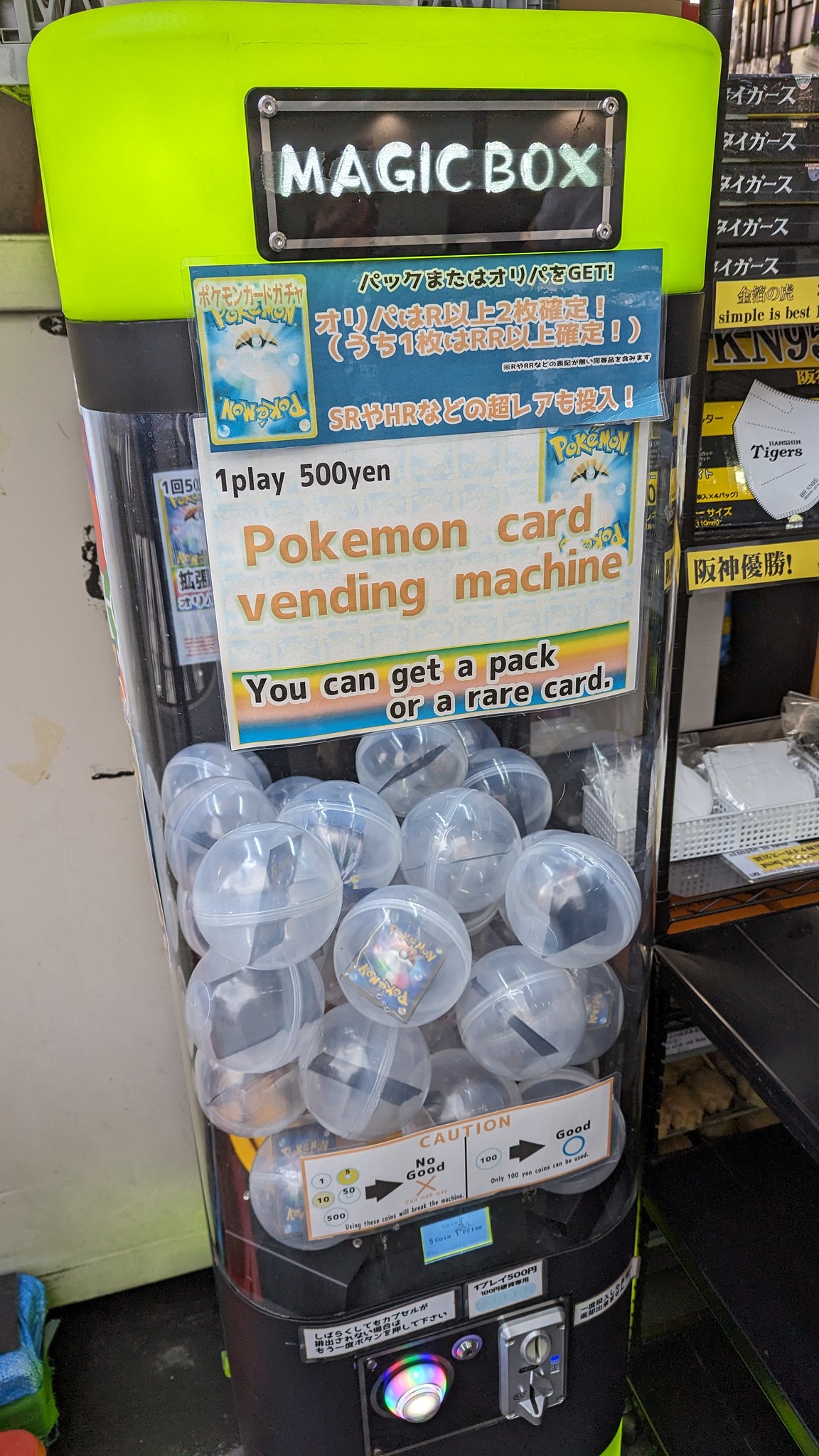This image captures a close-up view of a vending machine specifically designed for Pokemon card enthusiasts. The machine, adorned with a neon green top, prominently features a black box at the upper center with the words "Magic Box" displayed in bold, white letters. Below this, a large white sign reads "One Play 500 Yen Pokemon Card Vending Machine," indicating that for 500 yen, users can receive either a pack of Pokemon cards or a rare card. The vending machine's signage includes text in an Oriental language, adding an intriguing, international flair.

The transparent walls of the machine reveal its contents: giant plastic toy bubbles, each containing Pokemon-related items. Mounted on a three-tier stand beside the machine, you can observe more signage in what appears to be Chinese, with a combination of yellow and black lettering. At the base of the machine, clear instructions for usage are provided, along with an obvious slot for coin insertion, emphasizing its functionality. The entire setup suggests a playful yet intriguing experience for anyone eager to try their luck at obtaining a coveted Pokemon card.